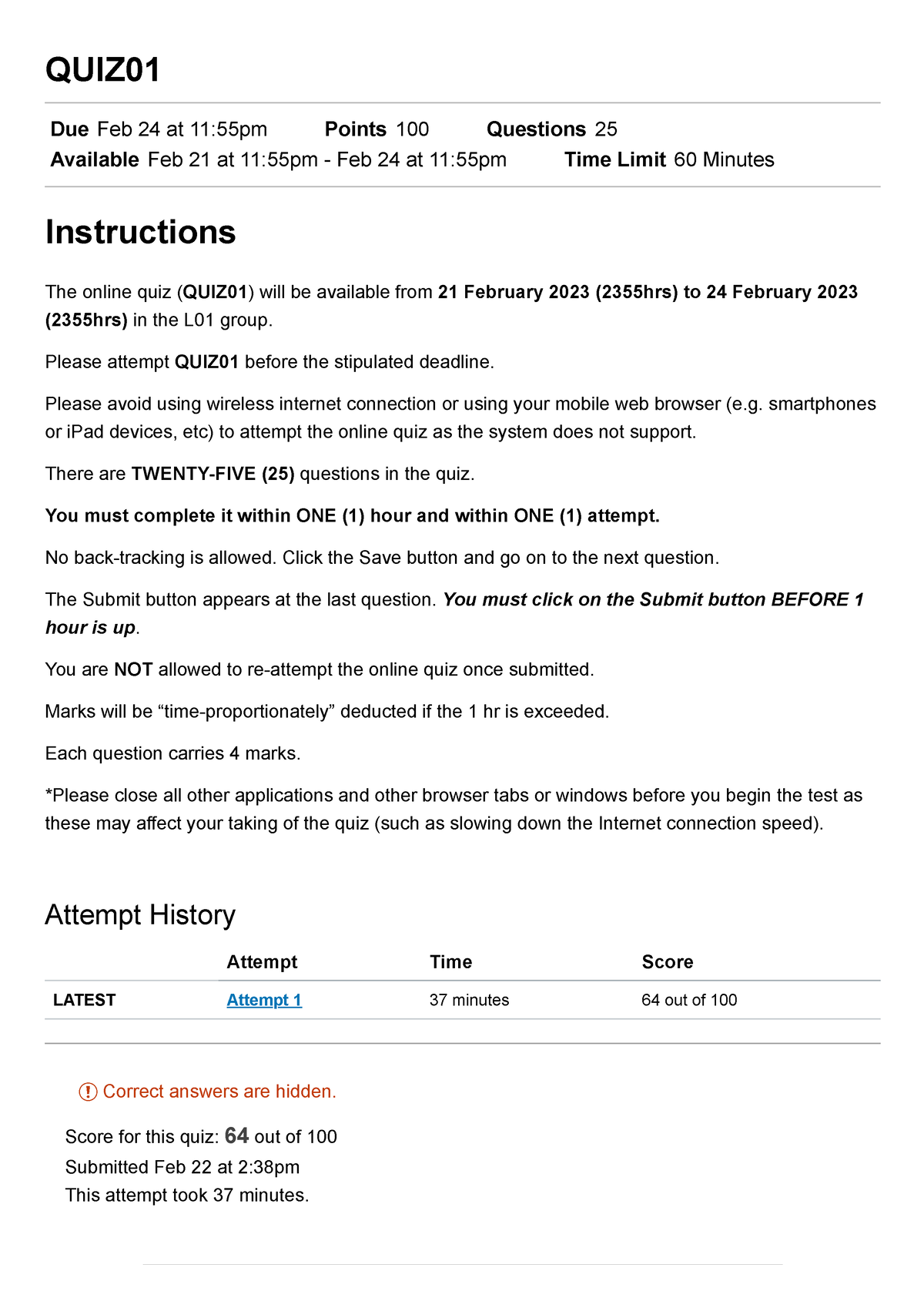A detailed photographic caption image showing a white page with black text detailing an online quiz schedule and instructions. The heading prominently reads, "Quiz 01 Due February 24th at 11:55 p.m." The following information is provided: 

- Points Available: 100
- Total Questions: 25
- Quiz Availability: From February 21st at 11:55 p.m. to February 24th at 11:55 p.m.
- Time Limit: 60 minutes

A large font heading marked "Instructions" states that Quiz 01 will be available to the L01 group from February 21, 2023, to February 24, 2023. It advises students to complete Quiz 01 before the deadline and warns against using wireless internet connections, mobile web browsers, smartphones, or iPad devices as the system does not support these setups. The quiz comprises 25 questions which must be completed within one hour and in one sitting, with no backtracking allowed between questions. Participants are instructed to save their progress and move on to the next question. 

At the bottom, the page displays the latest quiz attempt, labeled "Attempt 01" in blue, showing a score of 64 out of 100.